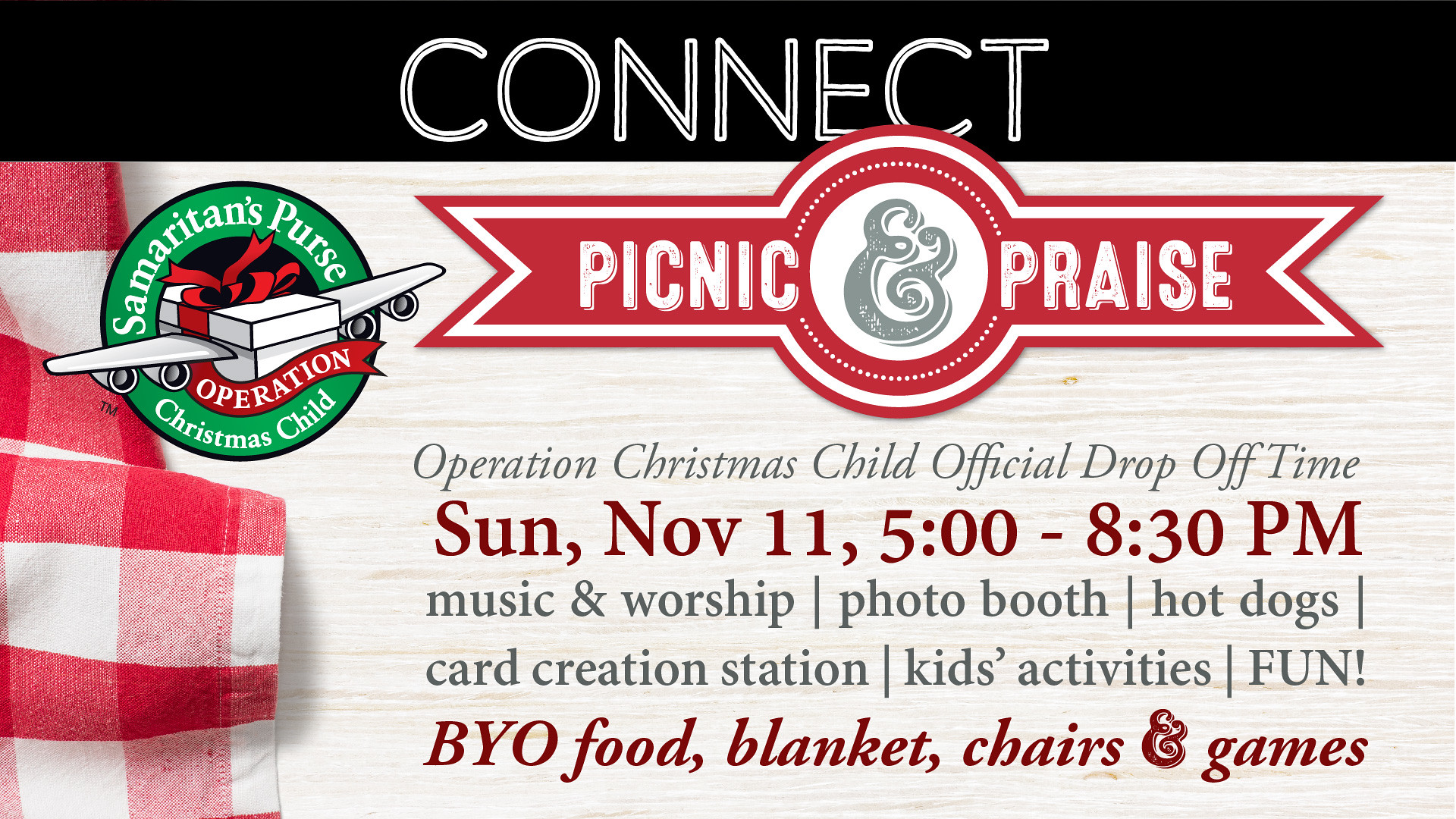This horizontal digital advertisement prominently features a black banner at the top with the word "CONNECT" in bold white capital letters. Below this banner, the background resembles light wood grain. On the left side lies a red and white checkered napkin, adding a picnic ambiance. To the left center, a green circle outlined in black displays the logo for "Samaritan's Purse Operation Christmas Child," featuring a white present wrapped with a red bow and airplane wings. Adjacent to it on the right, in elegant red script, reads "Picnic and Praise." Below these elements, the ad details "Operation Christmas Child Official Drop-Off Time: Sunday, November 11, 5:00 to 8:30 p.m." Attendees can look forward to "Music and Worship, a Photo Booth, Hot Dogs, a Card Creation Station, Kids Activities, Fun," and are encouraged to "BYO Food, Blanket, Chairs, and Games."